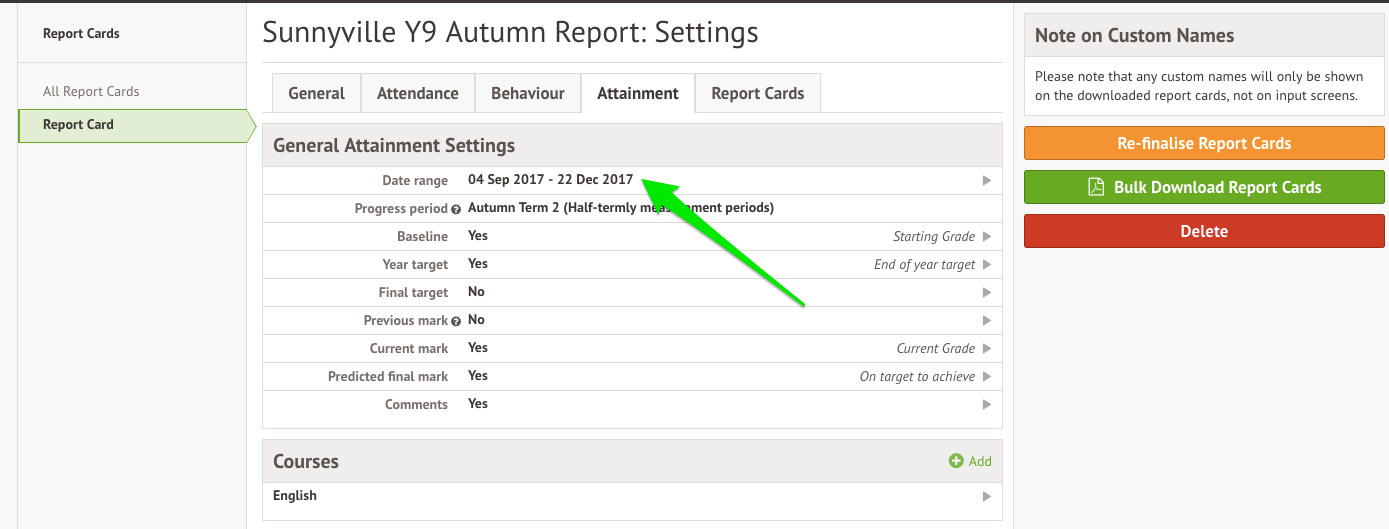The image depicts a grading report interface for Sunnyville School's Year 9 autumn term reports, specifically designed for managing and creating report cards. The interface features a left-hand menu with options such as General, Attendance, Behavior, Attainment, and Report Cards, with 'Attainment' currently highlighted.

Key details include:
- **School and Term Information:** "Sunnyville Y9 Autumn Reports and Settings"
- **Date Range:** From September 4, 2017, to December 22, 2017, highlighted with a large green arrow.
- **Progress Period:** Autumn Term 2, with baseline and target year options available.
- **Student Details Section:** Including fields for starting grade, end-of-year target, current grade, on-target status, final mark, and comments.
- **Courses Section:** Lists various subjects such as English, with an option to add more. It includes a column with options like "No to custom names".
- **Action Buttons:** To the right, there are buttons for finalizing report cards in orange, bulk downloading report cards in green, and deleting report cards in red.

This interface is not used for reading report cards but for the administrative tasks of creating and managing them.